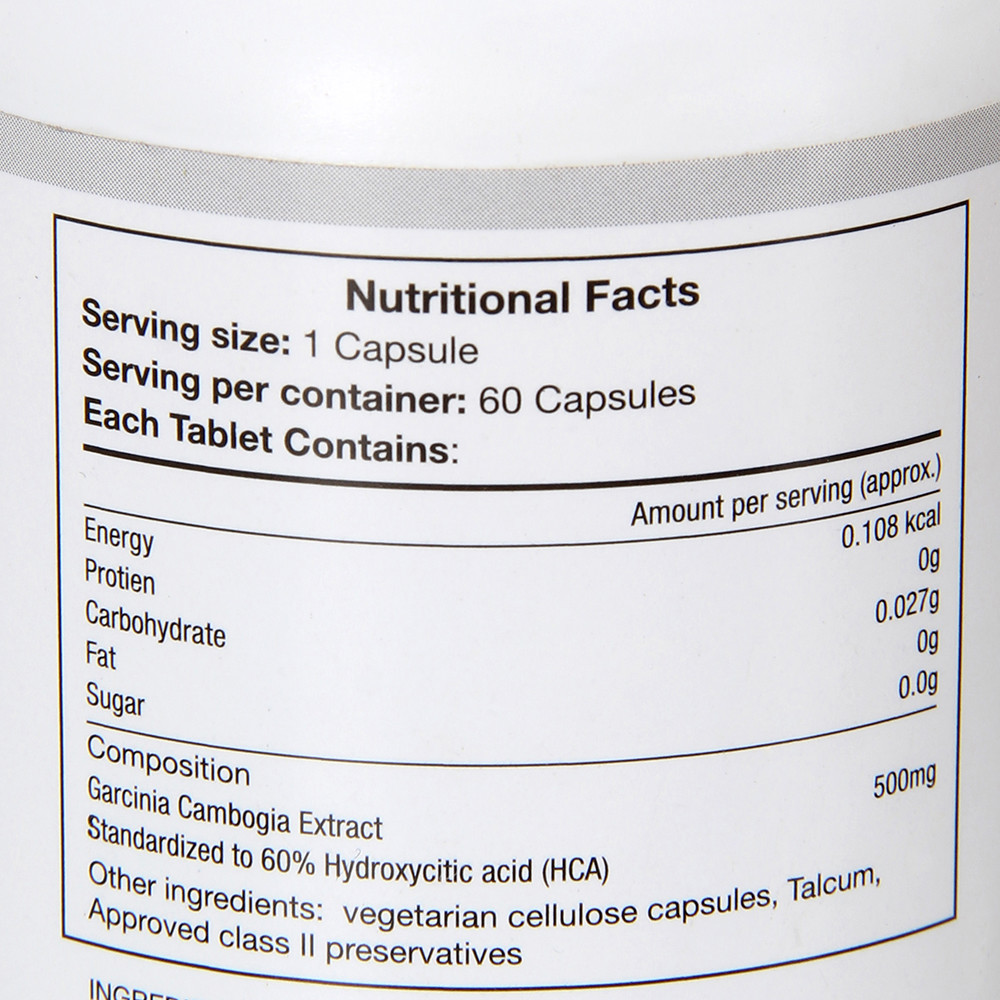This image features a detailed label on a white bottle or container, presenting the nutritional facts in black ink. The label indicates the serving size as one capsule, with each container holding 60 capsules. Each capsule delivers energy, protein, carbohydrates, fat, and sugar. It also lists the composition specific to Garcinia Cambogia extract, standardized to 60% Hydroxy Citric Acid (HCA). Additional ingredients include vegetarian cellulose capsules, talcum, and approved class 2 preservatives. This label is for a dietary supplement containing Garcinia Cambogia.